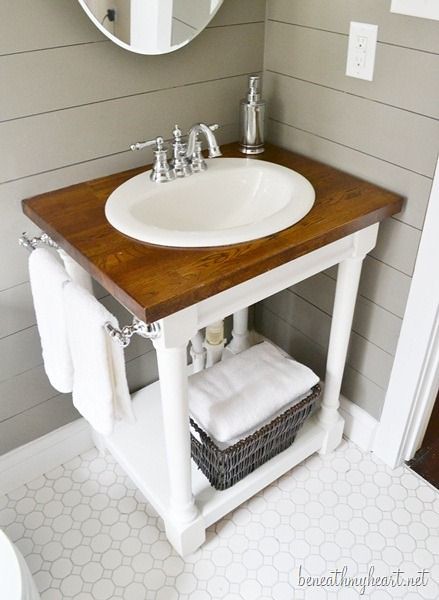This photograph showcases a charming bathroom vanity characterized by its open-bottom design, with exposed plumbing and spindle legs painted in a matching white. The vanity features a natural wood countertop with a surface-mounted sink that sits above the surface, accentuated by a bezel around its edges. A stylish high-arc, double-handled bathroom faucet graces the sink, complemented by a coordinating pump soap dispenser positioned in the corner.

The back wall is adorned with horizontally patterned gray tiles, adding a rustic yet refined touch to the space. An oval mirror with an edge that mirrors the sink's design is mounted just above the vanity, enhancing the cohesive aesthetic. To the right of the sink, a white outlet with a white outlet plate blends seamlessly into the decor.

The floor is a stunning mosaic of hexagon tiles, paired with a pristine white mop board that contrasts elegantly with the gray walls. Below the vanity, a wicker basket holds neatly folded towels, emphasizing both functionality and style. The exposed plumbing beneath the vanity is painted white to match the spindle legs, maintaining visual harmony.

To the left of the vanity, a towel rack holds two neatly hung towels, further contributing to the room's practicality and charm. In the bottom right corner of the image, the words "beneathmyheart.net" are discreetly displayed, hinting at the image's source.